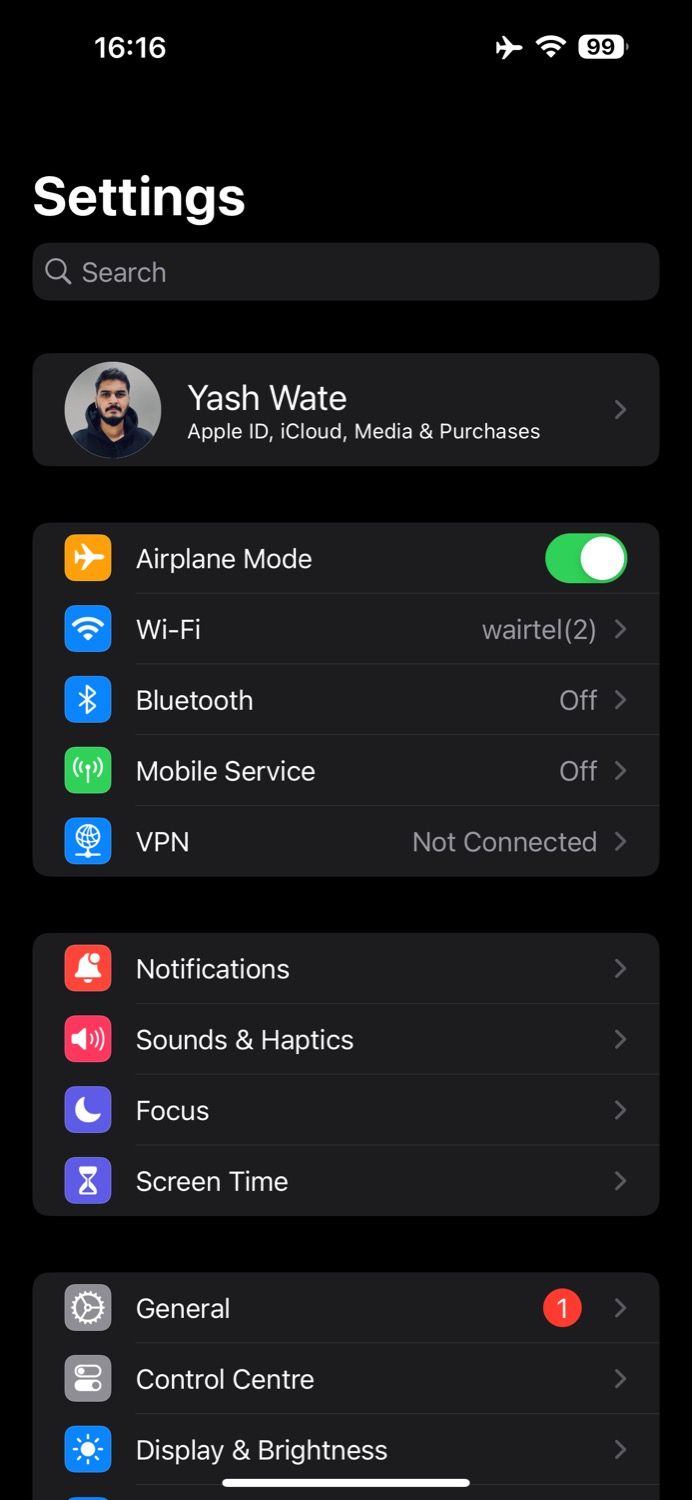A detailed screenshot of an iPhone Settings menu is displayed with a clean black background. At the top, centered in white lettering, is the word "Settings." Directly below, a search bar is visible. Beneath the search bar, the name "Yash Wate," with the spelling Y-A-S-H W-A-T-E, is shown. Adjacent to the name, to its left, is a profile picture. 

The section under the name includes links for "Apple ID, iCloud, Media & Purchases." Below this, the main menu items are listed, starting with "Airplane Mode," which is currently turned on. Following are the options: "Wi-Fi," "Bluetooth," "Mobile Service," and "VPN."

Proceeding to the next section, there are menu items for "Notifications," "Sounds & Haptics," "Focus," and "Screen Time." 

Under this, a new section starts with the heading "General," which has a red notification badge displaying the number 1 in white. The menu continues with "Control Center" and "Display & Brightness."

At the very bottom of the screenshot, a thin white line can be seen running horizontally across the center, representing the boundary of the menu.